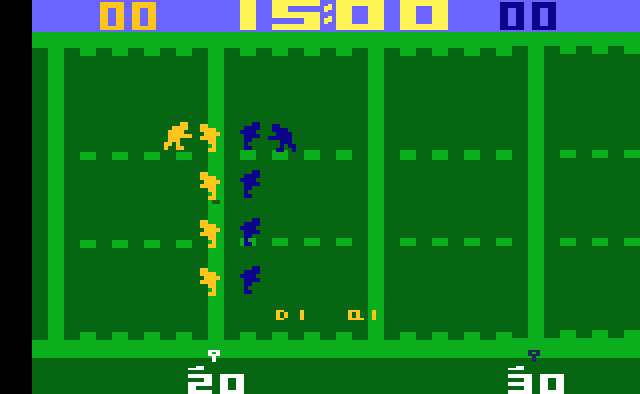This image is a screenshot of a computer game. On the left edge of the screenshot, there is a vertical black strip. Adjacent to this strip, at the top of the screen, is a rectangle filled with a periwinkle blue-purple color. Inside this rectangle, on the left, there are two orange block-shaped zeros positioned side by side. In the center of this rectangular area is a yellow block displaying the number "15," followed by two colons. To the right of the yellow block are two yellow zeros, and further to the right are two smaller black zeros in alignment.

Beneath this section is a dark green field, bordered at the top and bottom by horizontal green lines. This field features evenly spaced, vertical thick lighter green lines, and two dashed horizontal light green lines with a space in between. On the left side of the field, there are five green, square-shaped player avatars indicative of computer-controlled characters. To their right, there are five blue, square-shaped computer players positioned similarly.

At the bottom left of the screen, the number "20" is displayed in bold white block letters, while the bottom right corner shows the number "30," also in bold white block letters.